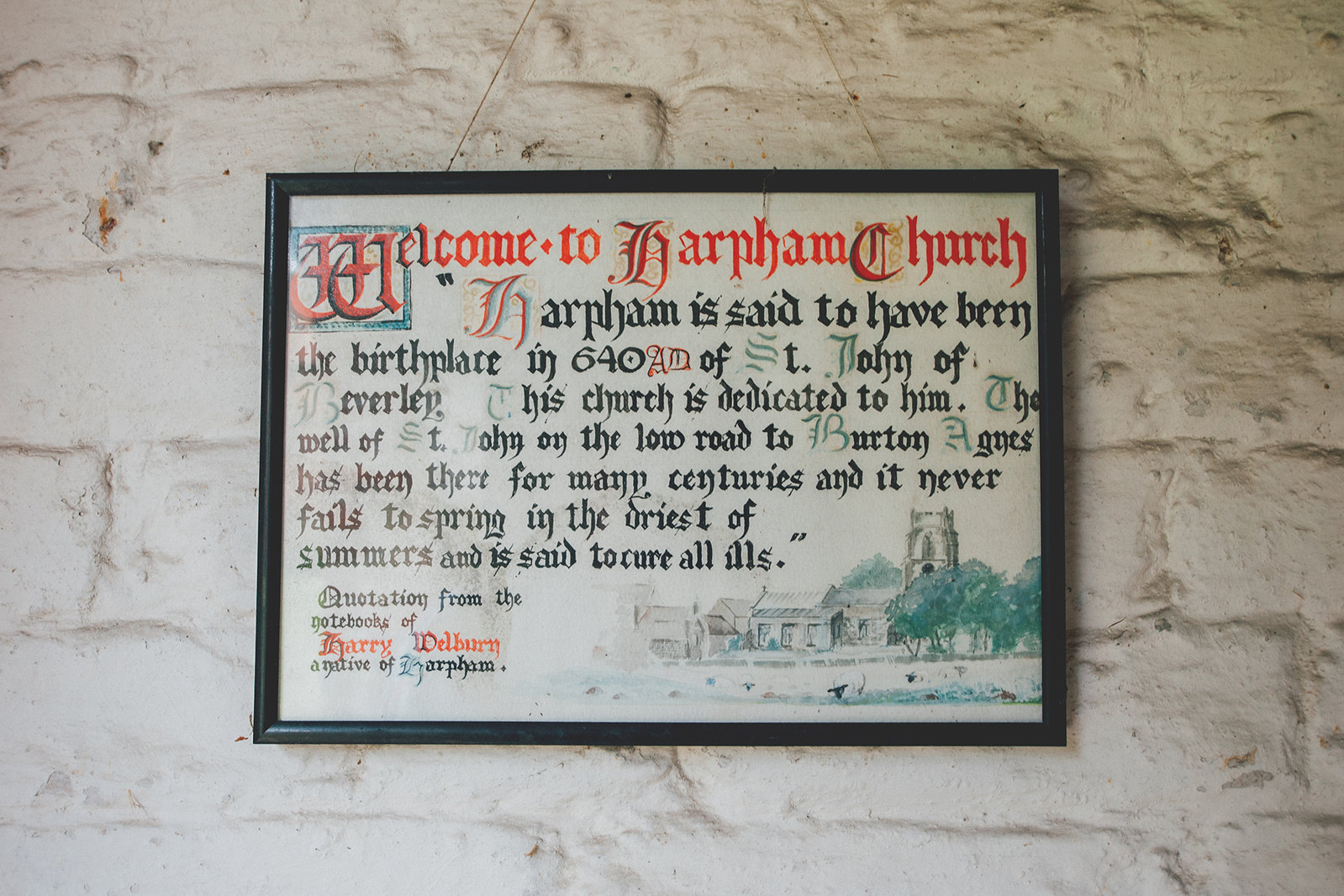The image depicts a framed plaque mounted on a white cement wall. The black frame encases a detailed inscription with specific stylistic features. At the top, in bold red text, it reads "Welcome to Darfam Church." The primary text of the inscription is in an old English type font, predominantly black, with significant portions highlighted in red. Notably, the first letter of the primary text and certain key elements such as "640 A.D." and the name "Harry Wellborn" are in red, adding emphasis. The plaque recounts that Darfam Church is said to have been the birthplace of St. John of Beverly around 640 A.D. The church is dedicated to him, and it mentions the St. John's well on the low road of Burton Agnes, a site renowned for never drying up and reputed to cure all ills. At the bottom left, there are quotations from the notebooks of Harry Wellborn, a native of Darfam, with his name also highlighted in red. The lower section of the plaque features a watercolor illustration of the church, adding a visual element to the historical narrative.